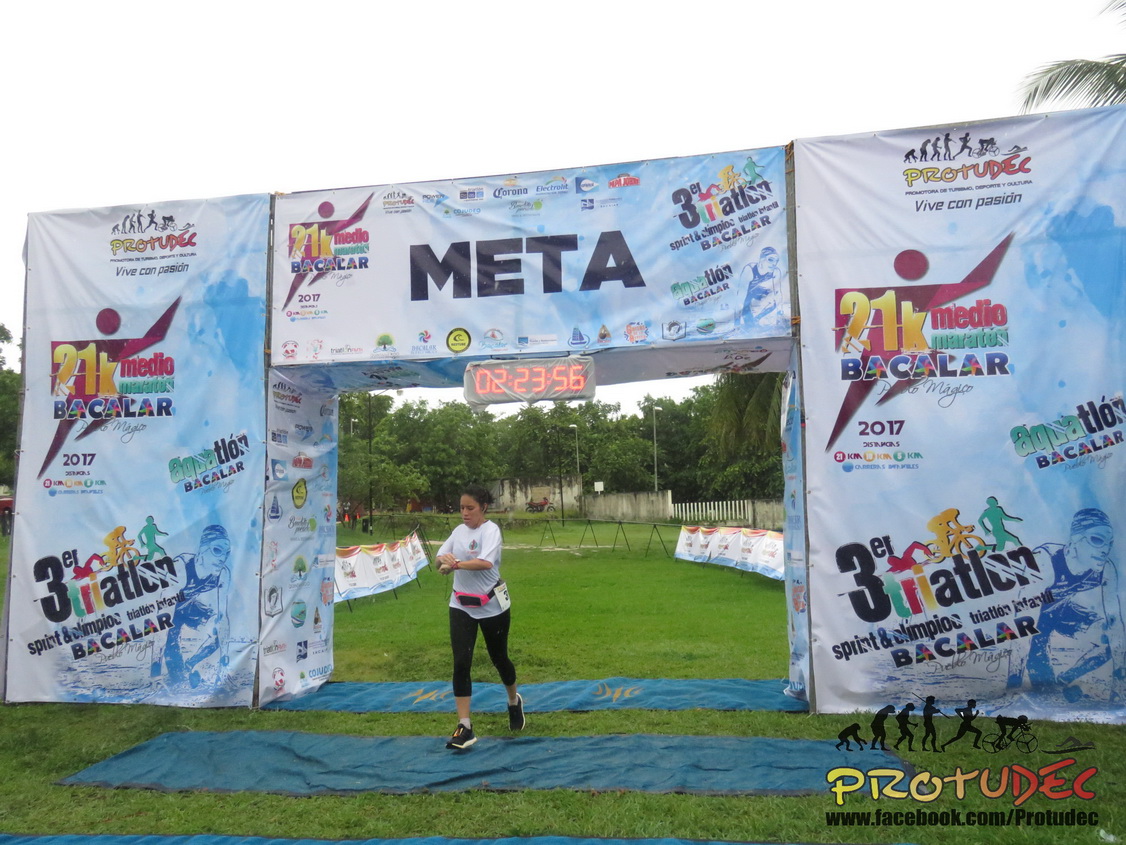A woman, dressed in a white shirt, black running pants, and black sneakers, has just crossed the finish line of a marathon race. The finish line, located in a grassy field, is marked by a large, arch-like scaffolding structure covered with a tarpaulin bearing various logos, including sponsorship images of bicyclists and the name of the marathon, 'Meta'. The event is identified as the 21k Media Marathon Bacalar 2017. Suspended from the center of the archway is a digital timer displaying 2 hours, 23 minutes, and 56 seconds. The woman, who also has a pink fanny pack, is looking at a watch on her left wrist, possibly to stop her timer. There is additional branding visible, including a logo reading 'Protudec' at the bottom right.